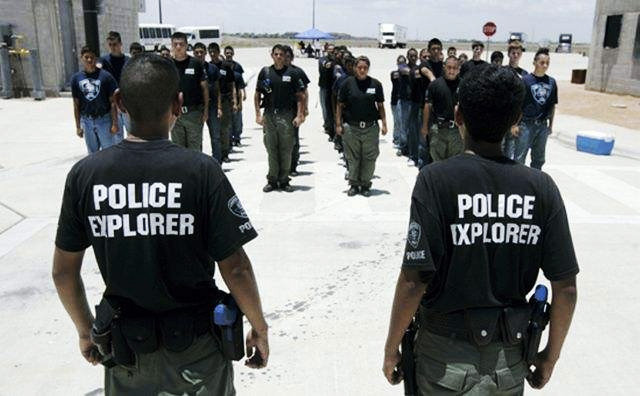The image captures a training session for police recruits in a cold, likely urban area, showcasing a rectangular, horizontal frame with snow on the ground. The backdrop features gray buildings and an overcast, gray sky. In the foreground, two men, with their backs to the camera, wearing black short-sleeved uniforms labeled "Police Explorer" in bold white text, stand prominently. These uniforms also feature badges near the sleeves and holstered guns at their hips. Facing them are several organized columns of approximately 20 to 30 recruits standing at attention. The recruits are dressed in black shirts, with some wearing dark blue shirts on the ends of the lines, paired with either green pants or blue jeans. The background reveals additional elements of the training setting, including white buses, semi-trucks, and various signs. The scene is set on a large concrete area, framed by concrete walls on either side, further emphasizing the structured, regimented nature of the training environment.